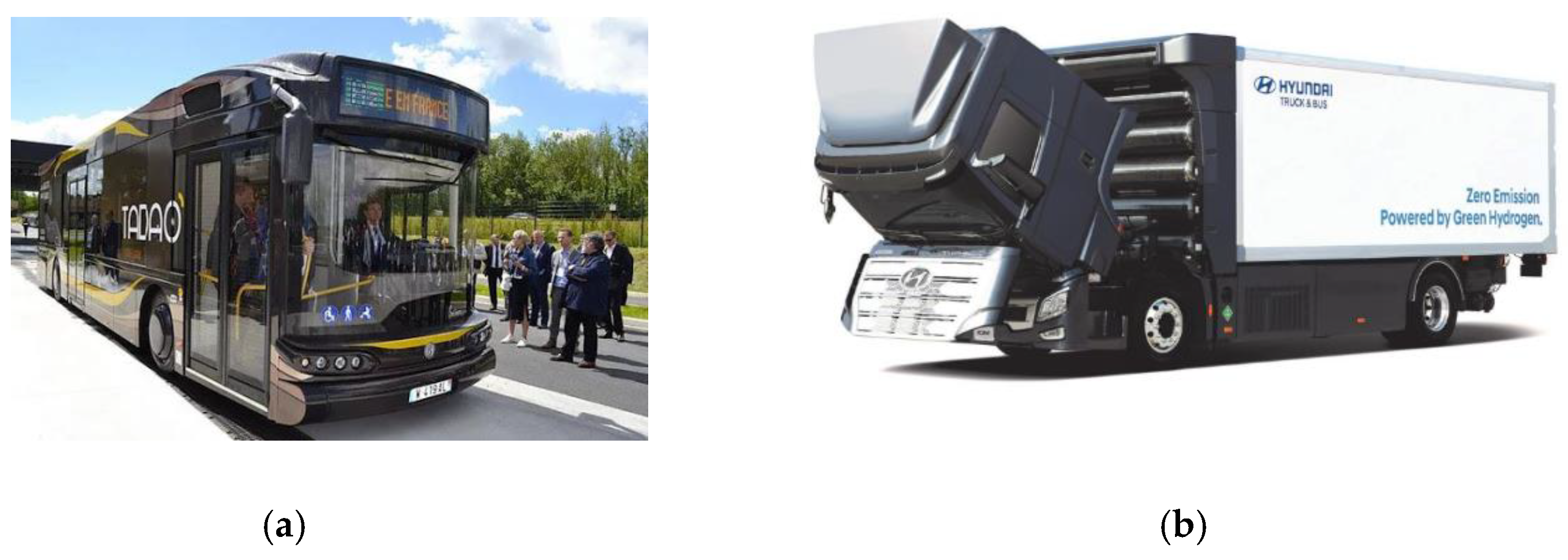The image is a landscape-oriented color photograph featuring two side-by-side pictures labeled (A) and (B) respectively. Picture (A) shows a dark gray charter bus with yellow markings along its body, including a yellow strip on the front. The bus appears to be stationary at the curb, facing the viewer at an angle, with several people standing on the road observing it. The sky is light blue with white clouds, and there are trees and fields in the background. The bus has "T-A-D-A-L" written on its side, indicating its possible destination. Picture (B) displays a white panel truck with its cab tilted forward, exposing a structure with hydrogen tanks behind it. The truck features the Hyundai logo and the phrase "Hyundai Trucks" on the top left corner, while the bottom right corner reads "zero emission powered by green hydrogen" in greenish-blue text.